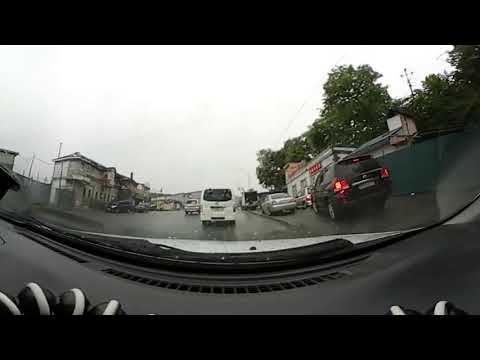This image is a still shot from a dash cam taken from inside a white car, identifiable by the visible hood at the bottom of the frame. The scene outside the windshield shows a wet, overcast day, suggesting recent rain under a cloudy sky. The road ahead features multiple lanes, lined with various vehicles. Directly in front of the car is a white minivan. To the right, a black SUV has its brake lights illuminated, followed by a silver car ahead of it. Several indistinct cars can be seen further down the road. The setting appears to be a poorer or older section of a small town, characterized by one to two-story buildings on either side of the street, some partially concealed by green leaf trees. The presence of power lines adds to the urban ambience. On the right side of the image, there is a green fence and a small white building with trees behind it. The windshield might be dirty or streaked with raindrops, enhancing the dreary atmosphere of the scene.